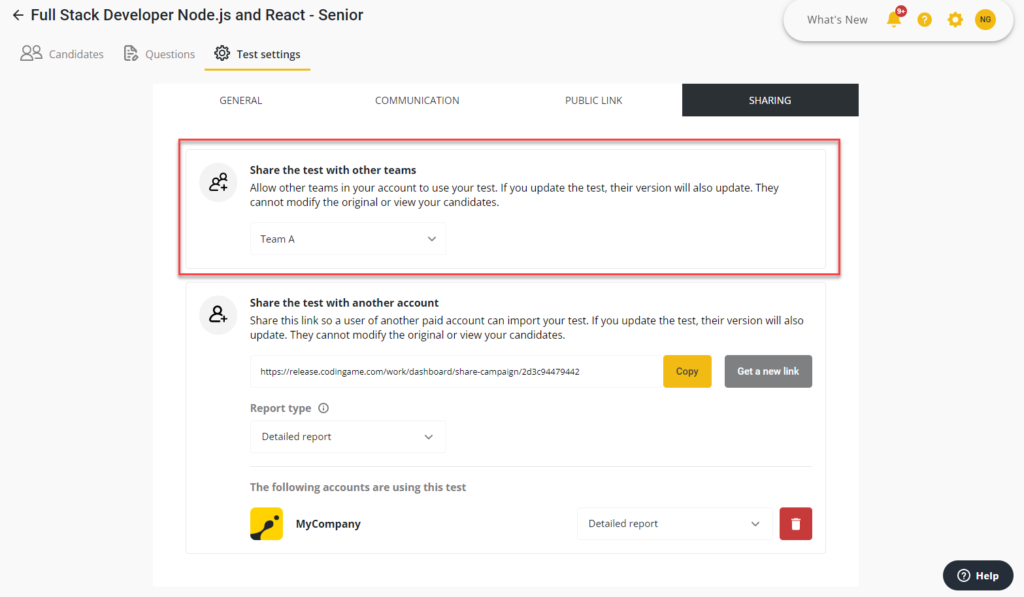This image is a cropped screenshot of what appears to be either an app or a web page, specifically a settings interface. The overall color scheme is primarily white, accented with shades of yellow, black, and dark gray. At the top of the page, the heading reads "Full Stack Developer Node.js and React Senior". Beneath this heading, there are three tabs labeled "Candidates," "Questions," and "Test Settings." The current view is on the "Test Settings" tab, which is highlighted with an underlining yellow line.

Within the "Test Settings" tab, there are additional sub-tabs: "General," "Communication," "Public Link," and "Sharing." The "Sharing" sub-tab is currently open, displaying several options and associated descriptive text. The two primary options are "Share the test with other teams" and "Share the test with another account," both accompanied by explanatory information. A red rectangular outline emphasizes the "Share the test with other teams" option.

At the bottom of the page, it states, "The following accounts are using this test," with "My Company" listed as the account. There is an option to select a detailed report, next to which is a red trash bin icon for deletion. In the bottom right corner, a black "Help" button is visible.

In the top right corner, four yellow icons are displayed: a notifications bell, a question mark, a gear (likely for settings), and a profile picture marked with the initials "NG." There is also a "What's New" button located near these icons.